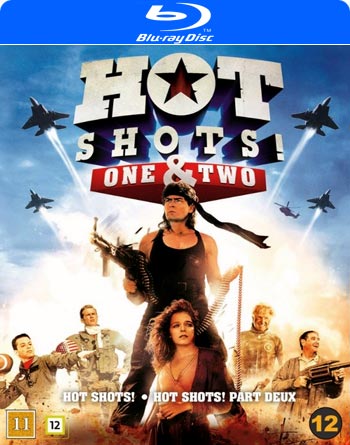The Blu-ray disc cover for "Hot Shots One and Two" features a striking movie poster with a detailed scene. Dominating the center is a light-skinned man wearing a black tank top, black headband, and dark pants. He stands confidently with a machine gun in his hands, the headband's tail flapping to the right. Directly below him stands a light-skinned woman with dark brunette hair, clad in an orange shirt and draped with a dark scarf over her left shoulder, reaching about his torso height.

Flanking the central duo are four men, two on each side, dressed in tan army fatigues. The background is a bright blue sky dotted with four fighter jets zooming in formation, two on each side of the title text.

Above the central figures, the title "Hot Shots" is prominently displayed in three-dimensional letters with a black outline, and below it, in white text, "One and Two" is highlighted in red. A blue horizontal strip across the top of the cover features the Blu-ray Disc logo in white. Additional text at the bottom middle of the poster repeats the title: "Hot Shots," "Hot Shots: Part Deux." In the corners, the numbers 11 and 12 appear on the bottom left, and the number 12 on the bottom right, completing the detailed design of this action-packed movie poster.